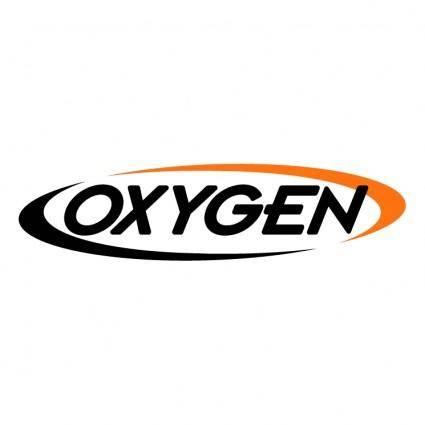The image showcases a digital close-up of a company logo centered against a completely white background. The logo features the word "OXYGEN" prominently in all capital letters, rendered in bold black text. Each letter is uniform in size and slightly slanted to the right, with particular design details such as the middle horizontal line of the 'E' extending minutely to the left and the 'G' having a squarish appearance at its end. Encircling the text is a thin, elliptical shape reminiscent of the Nike swoosh, with the left curve in black and the right curve in orange. This elliptical outline forms a pill-like enclosure around the word, with the right tip of the 'N' touching the orange curve. The swoops do not connect at their ends, leaving a small gap between their pointy tips, and the entire composition appears meticulously computerized, suggestive of a professional digital design.